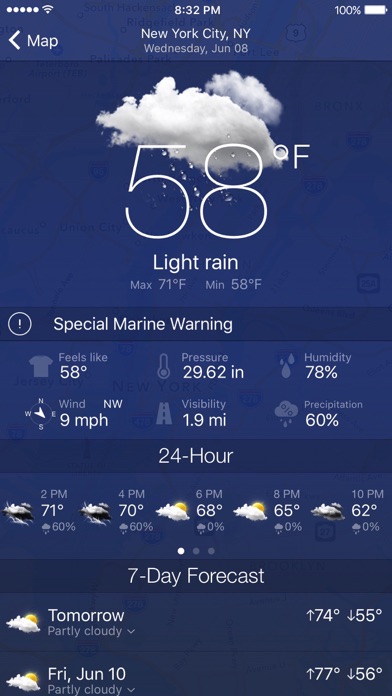Screenshot of a weather app displayed on a cell phone. 

At the top left corner, there are five round, filled-in white circles indicating full cellular signal. In the center, the Wi-Fi signal icon is displayed. The current time, 8:32 p.m., is shown next to it. On the top right, the battery indicator reads 100%.

Below, a white leftward arrow appears, possibly for navigation, labeled “Map” with each word capitalized. Centered is the title "New York City" with "NY" in uppercase. Just under it, the date "Wednesday, June 8th" is displayed. 

The background is blue with a white cloud and light rain icon, denoting the weather conditions. It reads "58°F, Light Rain," with a maximum temperature of 71°F and a minimum of 50°F.

A banner below contains an exclamation point inside a circle, noting a "Special Marine Warning" in white text.

Further down, another banner shows more detailed conditions:
- Feels like: 58°F
- Pressure: 29.62 inHg
- Humidity: 70%
- Wind: 9 mph NW
- Visibility: 1.9 miles
- Precipitation: 60%

A 24-hour forecast follows, with time intervals listed as 2 p.m., 4 p.m., 6 p.m., 8 p.m., and 10 p.m., showing different weather conditions and temperatures.

At the bottom, a 7-day forecast is displayed, starting with "Tomorrow" and "Friday, June 10th," indicating daily weather and temperatures on the right side.